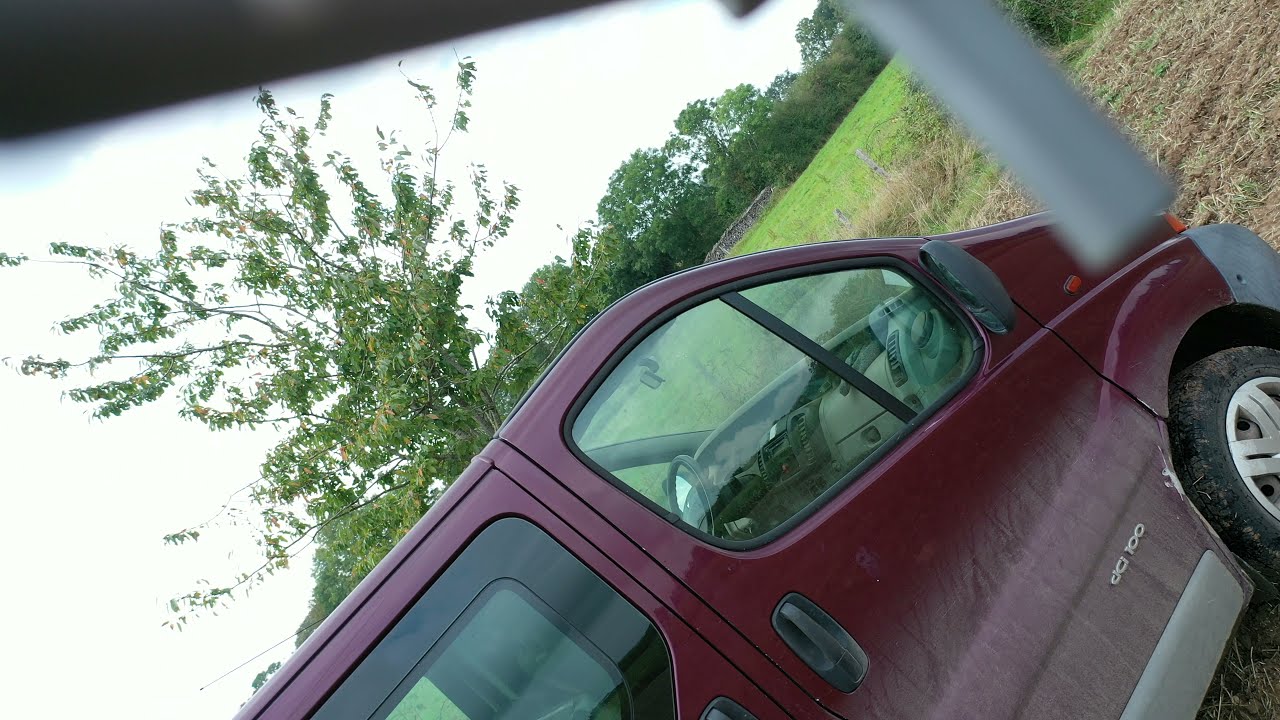The image depicts a slightly tilted maroon or burgundy minivan with a short nose, parked beside a house, visible along with part of a carport. The front passenger door and part of the sliding door are visible, showing significant dirt and white powder likely from rock salt. There is an illegible number on the bottom of the door. The van is parked in an area with overseeded grass covered in hay, amidst tall dead grass. The background features a green field, a rock wall, and a grove of trees, with one closer tree resembling a peach tree, all set under an overcast sky.